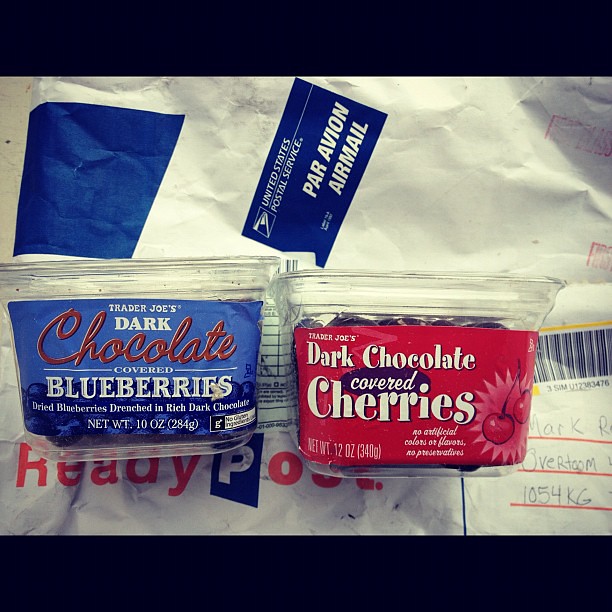The image depicts two clear plastic containers of Trader Joe's dark chocolate-covered fruits on their sides, displayed on top of airmail packages. The upper package features a blue box labeled "United States Postal Service" and "Par Avion Airmail" in white letters. The lower package, partially covered by the containers, is from ReadyPost with "Ready" in red letters and "Post" partly obscured by a blue box with white lettering. One container has a blue label that reads "Trader Joe's Dark Chocolate Covered Blueberries" with a cursive "Chocolate" and additional information about the product, including "dried blueberries drenched in rich dark chocolate, net weight 10 ounces (284 grams)." The second container has a red label with "Trader Joe's Dark Chocolate Covered Cherries," along with an image of cherries on the right. Below the containers, the package is addressed to "Mark R." and "S-VERTOOM 1054 kg," though the address is partially obscured. The setup suggests that these products were shipped to the recipient via airmail.